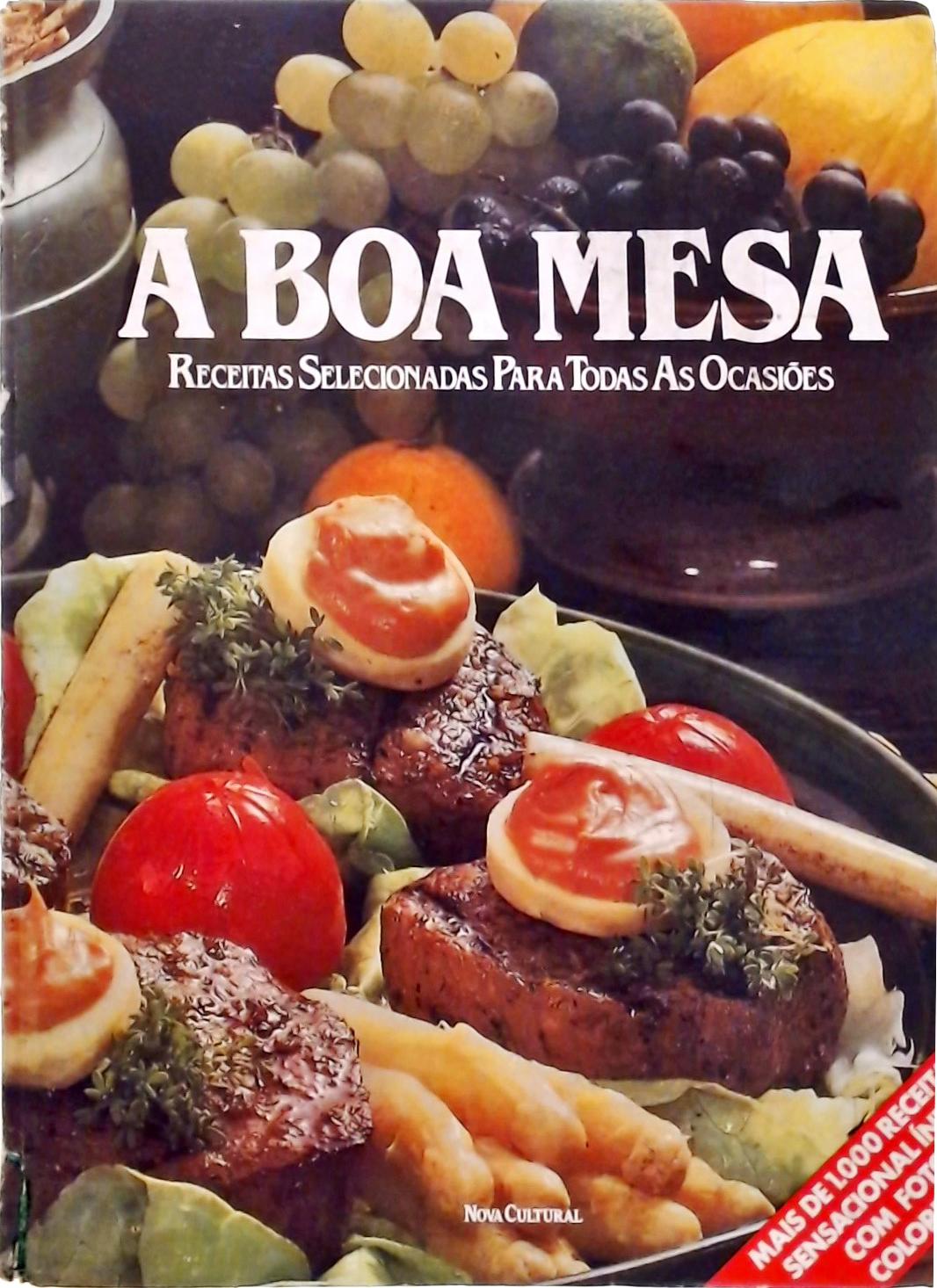The image appears to be the colorful cover of a cookbook, showcasing a vibrant display of various food items. Dominating the photo is a plate filled with a variety of foods, including cooked red meat, tomatoes, and a variety of green and yellow vegetables. Surrounding this plate, there are also an assortment of fruits such as green and black grapes, oranges, and potentially cinnamon sticks and breadsticks.

Across the top third of the cover, in large white capital letters, the title reads "A BOA MESA." Directly below this, in smaller white letters, the text reads "RECETAS SELECCIONADAS PARA TODAS LAS OCASIONES," suggesting the cookbook offers a wide range of selected recipes for all occasions. Just below this text is an image featuring more food items, enhancing the colorful and appetizing visual theme of the cover.

Towards the bottom of the cover, almost centrally positioned, the words "NOVA CULTURAL" are written in small white letters. Adding to the detailed design, a red diagonal band crosses the bottom right corner. Within this band, in white text, there are four lines: "MAIS DE 1000 RECEITAS," "SENSACIONAL," "COM FOTOS," and "COLOR," highlighting that the book contains over a thousand recipes, is sensational, and includes color photos. The cover, showing some slight wear on the edges, indicates it's a well-used and cherished cookbook.